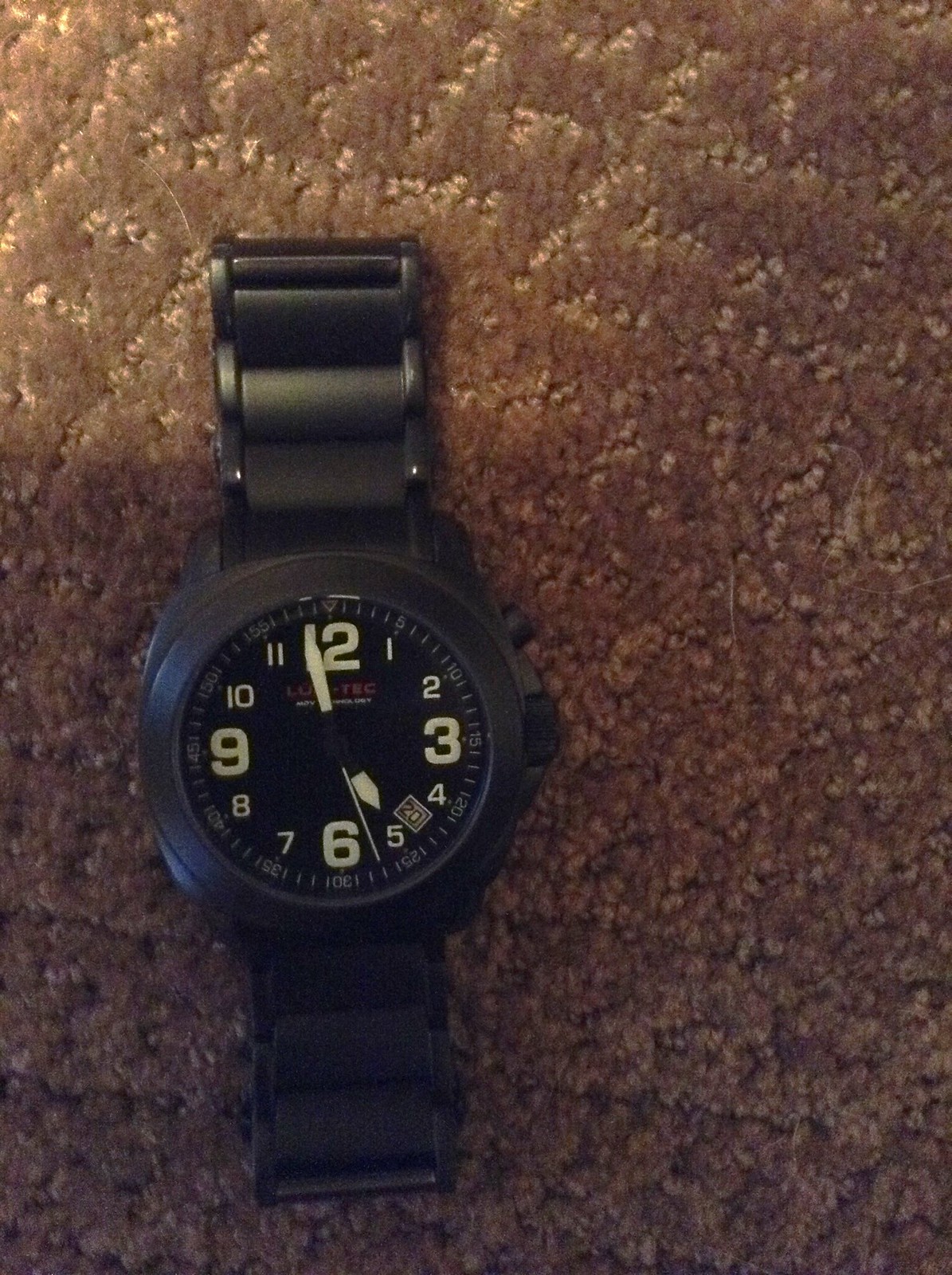This close-up image showcases a wristwatch resting on a thick, brown carpet. The watch features a stylish black chain-link band and a sleek black face. Prominently displayed on the face are large white numerals for the 12, 3, 6, and 9-hour markers, while smaller white numerals mark the remaining hours. Between the 4 and 5 positions, a small rectangular window reveals the date. The watch indicates that the time is precisely five o'clock, with the white second hand positioned between the 5 and 6 markers. The thick carpet beneath the watch appears to have some missing fibers in the top-left corner of the photograph, adding a touch of texture and imperfection. The watch itself is placed slightly to the left within the frame, creating an asymmetrical and visually interesting composition.